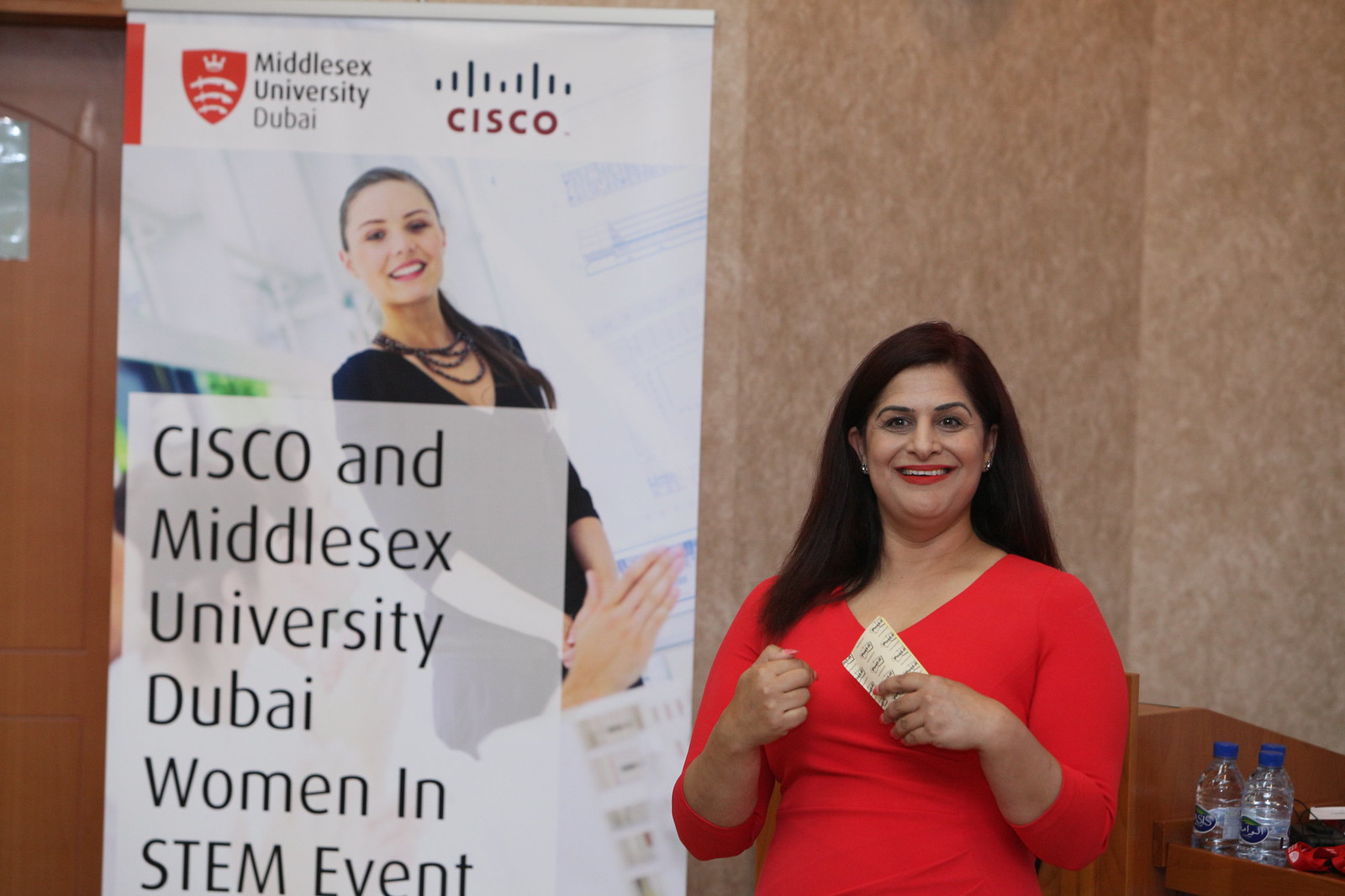This detailed photo captures a woman with long dark hair smiling warmly at the camera, her red lipstick enhancing her smile. She is dressed in a long-sleeved, red blouse and accessorized with earrings. The smiling woman is holding what appears to be notepads or papers in her left hand, positioned in front of her. To her right, a table with water bottles and other items is partially visible, including a red, indiscernible object.

She stands in front of a large white backdrop that prominently features the text "Cisco" and "Middlesex University Dubai," highlighting the event's title: "Cisco and Middlesex University Dubai Women in STEM event." This indicates the photo is taken at an event aimed at encouraging women in Dubai to pursue careers in science, technology, engineering, and mathematics (STEM). The setting appears to be inside a college room, further emphasized by the brochure beside her displaying another smiling woman's image. The background includes beige and brown walls, adding context to the indoor, academic environment.